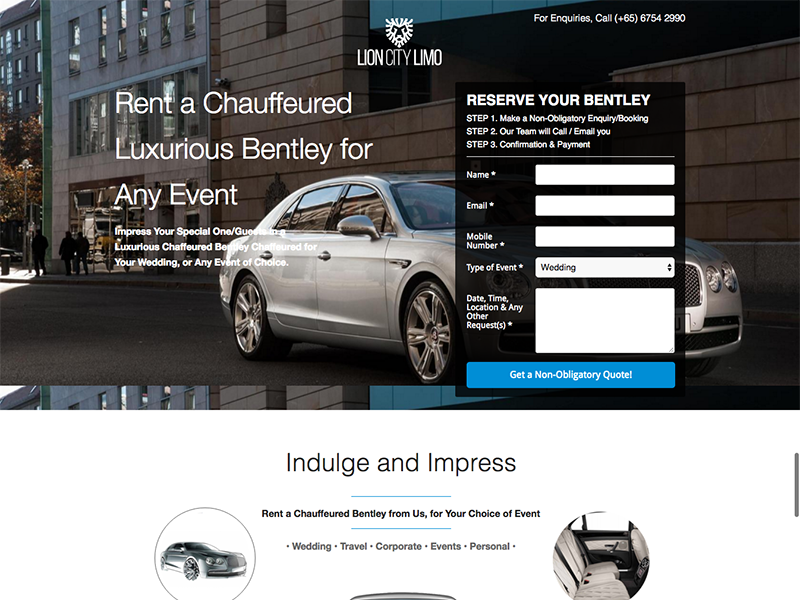A screenshot from a limousine rental company's website showcases their premium services. The top of the image displays the company's logo: "Lion City Limo" accompanied by a uniquely designed lion icon. Below this, a call-to-action line includes a contact number for inquiries. The cover image features a sleek, gray luxury sedan that resembles a limousine, prominently displayed against a bustling street backdrop. The car's polished exterior gleams, contrasting with the darker, busier backdrop where pedestrians can be seen. 

Overlaid text promotes the company's exclusive offering: "Rent a chauffeured luxury Bentley for any event." A brief description follows, encouraging clients to "Impress your special one/guests at your wedding or any event." An embedded form prominently located over the car image invites customers to "Reserve your Bentley," requiring details such as name and email to proceed. 

Beneath this section, on a white background, the phrase "Indulge and Impress" is visible, accompanied by a series of icons, suggesting additional features or services provided by Lion City Limo.